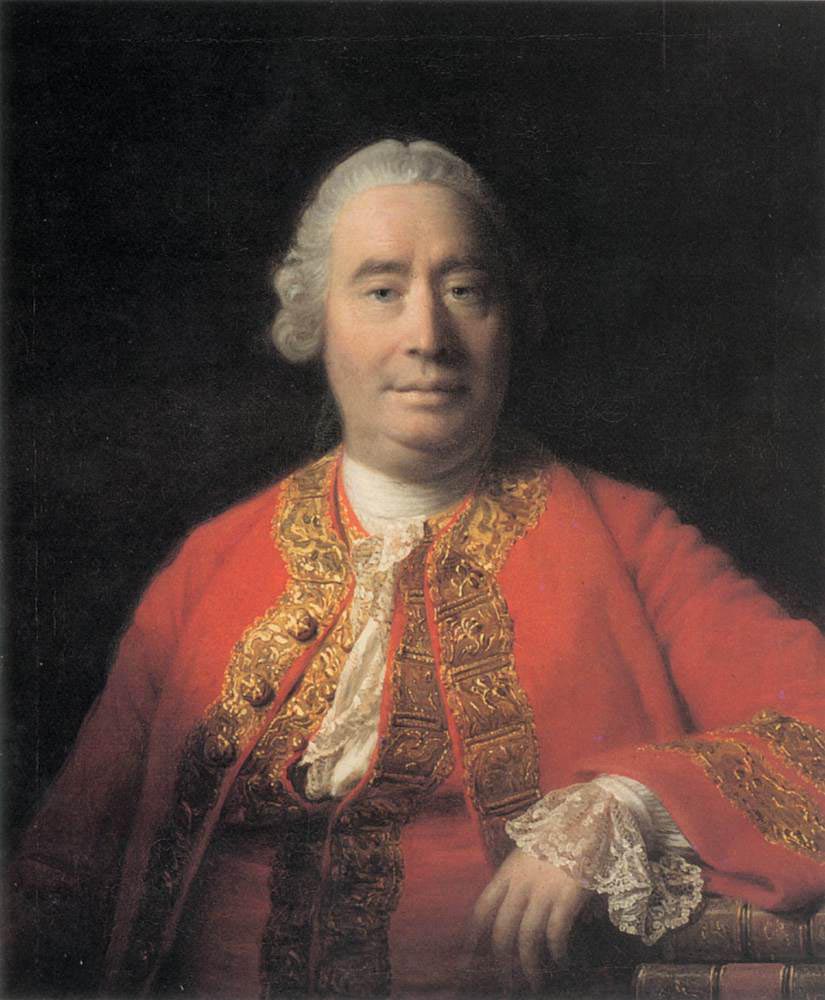This highly detailed and realistic painting depicts a somewhat plump European Caucasian man from the late 1600s to early 1700s, rendered from the torso up in a tall rectangular format. The background is predominantly black with faint gray etchings and undertones, creating a stark contrast to the subject. The man's light beige skin, double chin, and calm, neutral expression are finely detailed, with his blue eyes and a light gray powdered wig adding to the period accuracy. He wears a multi-layered, ornate outfit: the outer layer is a deep orange-red jacket with gold embellishments and large buttons, complemented by a similarly colored vest underneath, adorned with intricate gold embroidery. A white, lacy frock peeks through, and his left elbow rests on a stack of brown books, with his lacy cuff prominently displayed. The light falls softly from the right, highlighting the delicate textures and fine brushwork that make the painting remarkably lifelike.